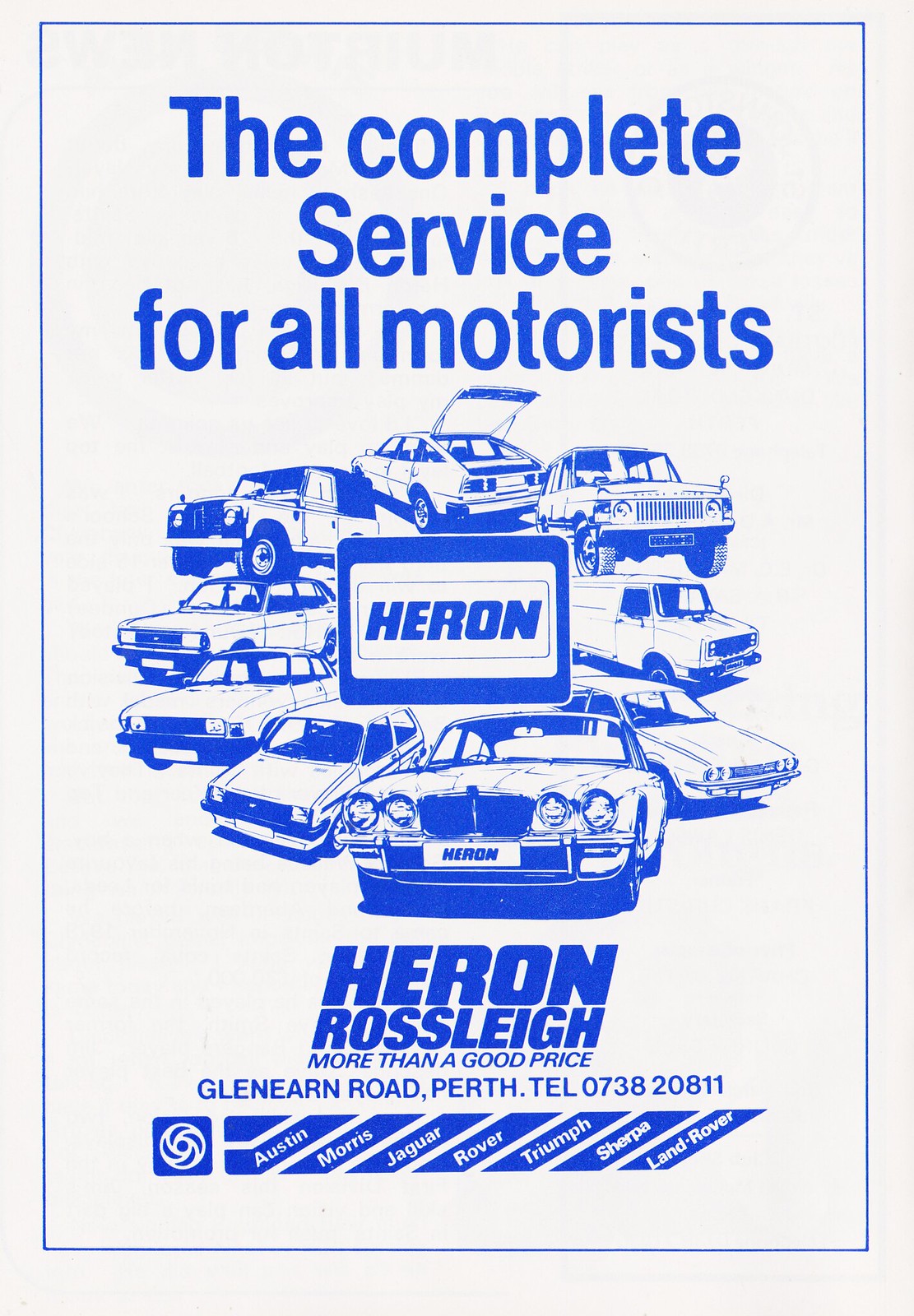This vertical rectangular poster is an advertisement for Heron, an automotive service company. The design, primarily in blue and white, has a thin blue stripe framing the text and a surrounding white border. Dominating the center is an image featuring various types of cars—including sports cars, SUVs, sedans, vans, trucks, and notably a Jaguar—all arranged in different directions around a blue-bordered rectangle with the word "Heron" prominently displayed. At the top, the poster reads, "THE COMPLETE SERVICE FOR ALL MOTORISTS" in large blue capital letters. Beneath the image, it states "HERON ROSSLEY, MORE THAN A GOOD PRICE" followed by the address "Glenirne Road, Perth, Australia" and a telephone number. The poster additionally features logos at the bottom, including names such as Austin, Morris, Jaguar, Rover, Triumph, Sherpa, and Land Rover, indicating the range of vehicles they service. Despite its slightly faded appearance, the piece retains a clear and concise blue and white monochrome aesthetic, reflective of an older, classic advertisement style.